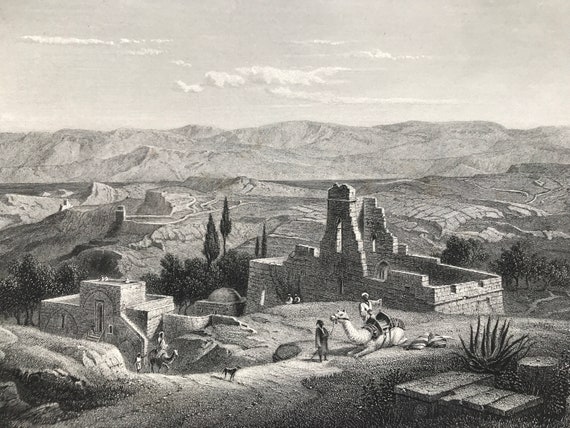This detailed black and white pencil drawing, reminiscent of old book illustrations, portrays a rugged Middle Eastern landscape. In the background, a vast mountain range stretches beneath a mostly clear sky, evoking a sense of Afghanistan or Iraq's barren terrain. The scene is set on a hillside overlooking a deep valley, with angular, square buildings crafted from stone. Notably, a small stone house stands in the right foreground, next to a larger, partially ruined fortress whose jagged walls and open windows suggest decay. In the immediate foreground, a camel sits placidly on the ground while a dark-robed man holds its ropes. Nearby, to the left, a trail descends the mountain, where another camel is ridden by a person with another walking behind. The bottom right corner includes wood planks next to a tree stump and a cactus or aloe plant. Additionally, a small dog observes the scene. The drawing captures a timeless, serene moment in a harsh, yet beautifully desolate environment.